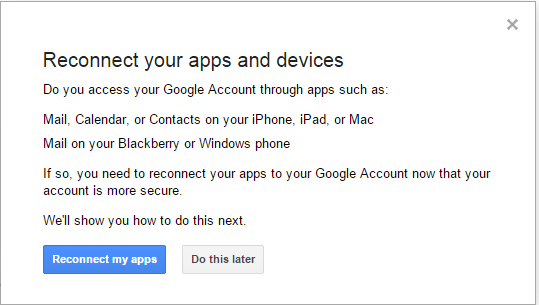The image is a screenshot of a notification message from Google. It features a simple white background with a light gray box in the center, which has a light gray 'X' in the top-right corner. The message content is aligned to the left and presented in a clean, black, Arial-like font. The title, "Reconnect your apps and devices," is bolded with the letter 'R' capitalized.

The message reads:
"Do you access your Google Account through apps such as Mail, Calendar, or Contacts on your iPhone, iPad, or Mac?
   Mail on your BlackBerry or Windows Phone?
If so, you need to reconnect your apps to your Google Account now that your account is more secure. We'll show you how to do this next."

Below the text are two action buttons: a blue button with white text that says "Reconnect my apps" on the bottom-left, and a light gray button with black text that says "Do this later" to the right of it.

The notification serves as a prompt to users, instructing them to reconnect their various applications and devices to their Google Account for security reasons.